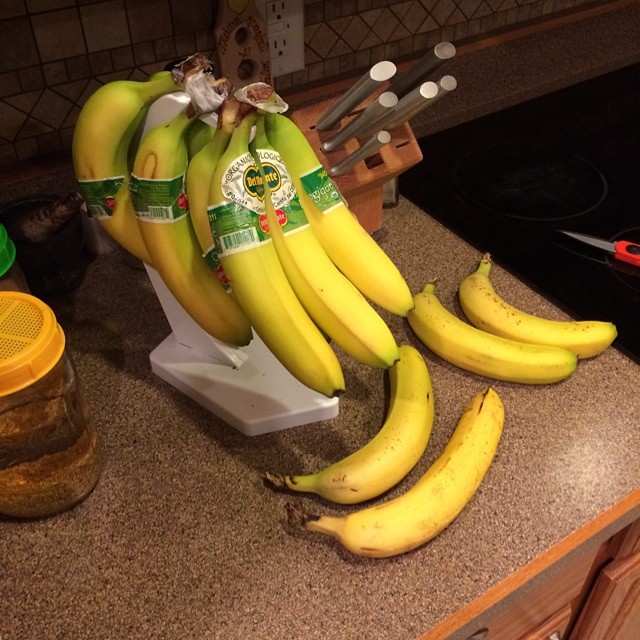A detailed color photograph taken from above captures a brown and black speckled granite kitchen counter with light brown wooden drawers beneath. Centered on the counter is a white banana hanger holding three bunches of bananas adorned with green Del Monte labels, some of which are slightly greenish at the tips but mostly yellow. Four riper bananas with brown spots lie separated on the counter below the hanger. To the left of the bananas, there's a clear jar about three-quarters full with a colorless liquid and topped with a yellow lid featuring holes. To the right stands a wooden knife block holding five stainless steel knives with silver handles, with a couple of empty slots visible. Adjacent to the knife block is an electric stovetop with a short knife featuring an orange handle placed on it. In the background, a textured brown wall with various shaped tiles and a white power outlet is visible.